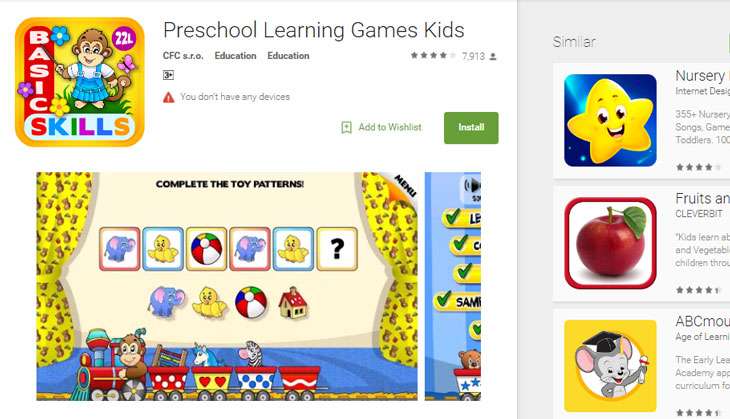This image is a screenshot of a desktop version of an app store page, though it's unclear whether it's from the Apple App Store or Google Play. The page showcases the app "Preschool Learning Games for Kids," which has a rating of 4 out of 5 stars based on 7,913 reviews. The app icon is a square with a yellow background and rounded edges. It features the word "Basic" written vertically on a red rectangle, and the word "Skills" horizontally on a white rectangle, with each letter in a different color (red, blue, green, purple, and yellow). Additionally, there's a cartoon image of a teddy bear in a white T-shirt and blue jumper.

Below the app icon, there is an image from the game that appears to depict a stage setup. Another image below this shows another teddy bear, this one dressed as a train conductor, riding a red train. These graphics are designed with a cute and colorful cartoon style.

On the right side of the screenshot, partially cut off, is a section titled "Similar" against a gray background. This section displays three app icons. The first icon is a gold star with a face; the second is a photographic image of a red apple; and the third is a cartoon character of a mouse wearing a graduation cap.